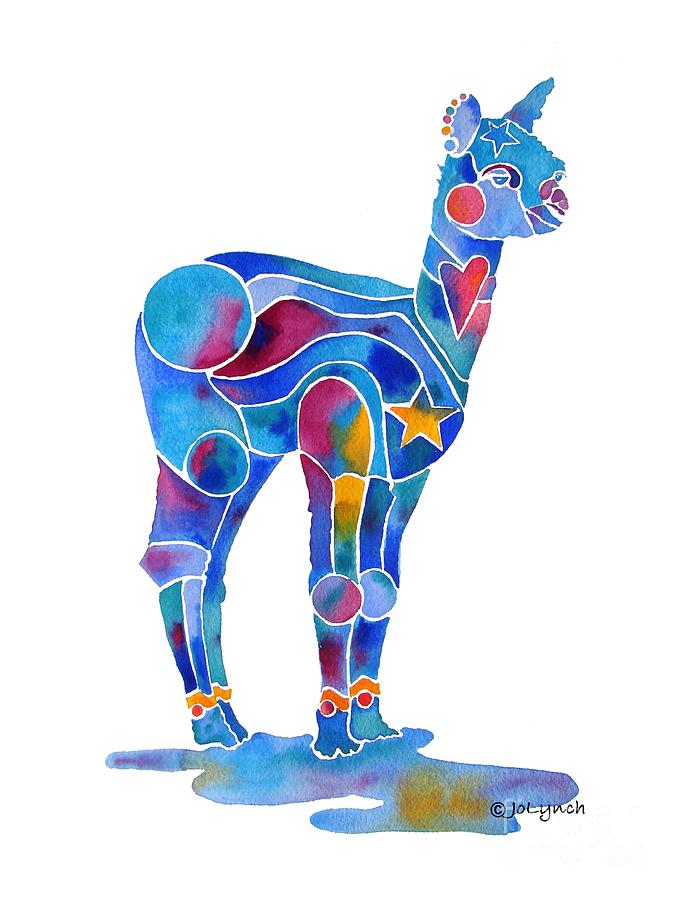The image depicts a highly stylized and colorful painting of a llama, created in a watercolor style and signed at the bottom right-hand corner by the artist, possibly J.O. Lynch, with a copyright symbol. This whimsical llama stands against a white background without any additional scenery. The llama features a vibrant mix of colors, predominantly blue, red, yellow, and green. Its body is adorned with various shapes and symbols: a blue star on its forehead, a large red circle on its cheek, a heart on its neck, and another star near its front shoulder. The knees of the llama are marked by round circles, and its ankles are highlighted with yellow anklets, which have small red balls beneath them. The composition includes white lines that form different shapes and ridges across the llama’s body. Beneath the animal is a colorful shadow or splash, incorporating shades of dark blue, light blue, yellow, and red. The entire painting is highly decorative and abstract, showcasing a lively and imaginative interpretation of a llama.